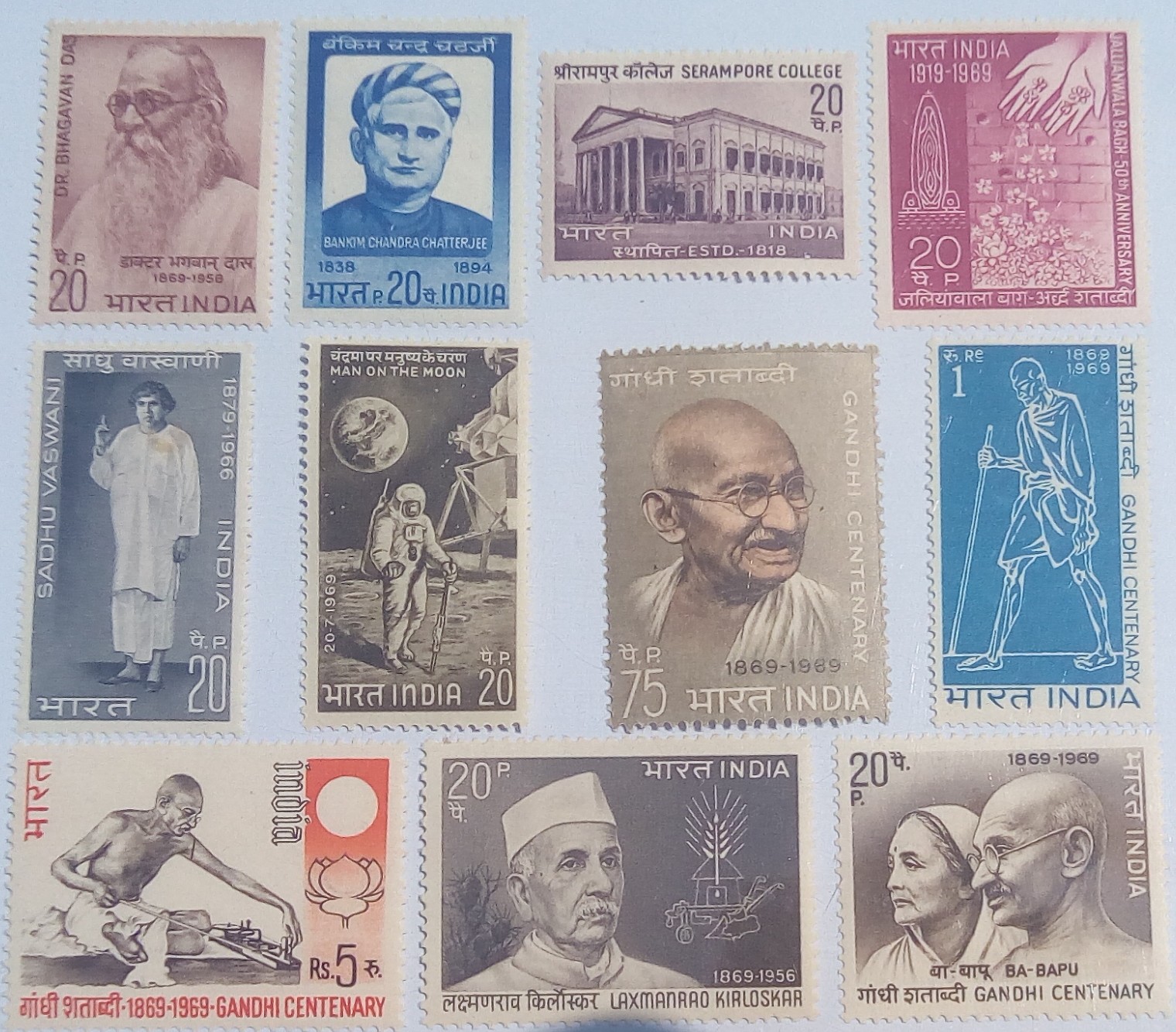The image showcases a meticulously arranged collection of twelve Indian postage stamps, displayed against a light blue background. The stamps are organized into three rows, with four stamps in each of the top two rows and three stamps in the bottom row. Each stamp features distinctive details, all tying to Indian heritage and history.

In the top row, the first stamp depicts Dr. Bhargavan with his glasses and long beard, labeled "20 pence, India". Next is a portrait of Banam Chandra Chatterjee (1838-1894) wearing a turban, also marked "20 pence, India". The third stamp showcases Serampore College with an image of a building and "20 pence, India". Lastly, a pink stamp commemorates the 50th anniversary of the birth of Jalamawara, illustrating hands dropping flowers (1919-1989) and marked "20 pence, India".

The middle row starts with a stamp featuring Sadhu Raswani (1879-1966) in a white outfit, labeled "20 pence, India". Following this is a black-and-white stamp of an astronaut on the moon, simply titled "Man on the Moon" and "20 pence, India". The next two stamps in this row honor Mahatma Gandhi: the first one, "Gandhi Santana 1869-1989", portrays him in his robe and glasses, priced at 75 pence, while the second one, a blue and white graphic, depicts Gandhi walking with a stick, marked "Gandhi Santana 1869-1969" and "20 pence, India".

The bottom row begins with another black-and-white image of Gandhi, this time making his own clothes, marked "Gandhi Santana 1869-1969" and "5 pence, India". Adjacent to this is a grey and white stamp of Lakshmanrao Kirloskar (1869-1956), inscribed with "20 pence, India". The final stamp in the collection features Gandhi alongside a woman, likely his wife, both wearing traditional attire, labeled "Gandhi Santana 1869-1969" and "20 pence, India".

Overall, the stamps exhibit vibrant colors including hues of blue, pink, grey, and orange, each narrating a piece of Indian history and cultural legacy.